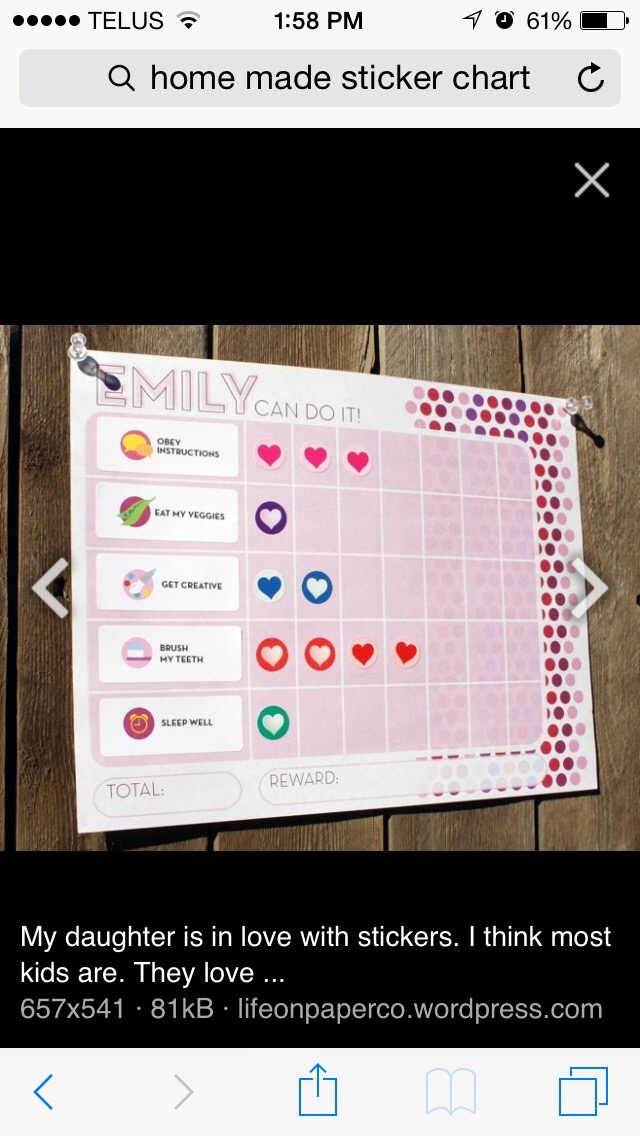This screenshot features an image that appears to be part of a series, captured from a computer screen, suggested by the interface elements visible at the top. The upper section includes a thick black bar with an X symbol in the right corner and a faint gray search bar above it. There are details like the time (1:58 PM), battery life (61%), various symbols, and the letters "T-E-L-U-S" indicating a network connection.

The main focus of the image is a "sticker chart" pinned against a light brown wooden wall background. The chart, with prominent pink text at the top proclaiming "Emily can do it," is divided into various tasks for which Emily earns stickers, a motivational tool typical for young children. The tasks and their corresponding stickers are as follows:
- "Obey instructions" with three red heart stickers.
- "Eat my veggies" with one red heart sticker.
- "Get creative" with two red heart stickers.
- "Brush my teeth" with four red heart stickers.
- "Sleep well" with one red heart sticker.

At the bottom of the chart, there are sections labeled "Total" and "Reward," both currently left blank.

A black bar beneath the image has text in white, stating: "my daughter is in love with stickers. I think most kids are. They love..." followed by an ellipsis. Below this, in gray, it reads "lifeonpapercode.wordpress.com." Other elements such as file size and additional navigation symbols for browsing or downloading further content are also visible near the bottom bar.

This detailed descriptive caption consolidates both observations, giving an elaborate overview of the screenshot and its contents, highlighting recurring themes and shared visual elements.